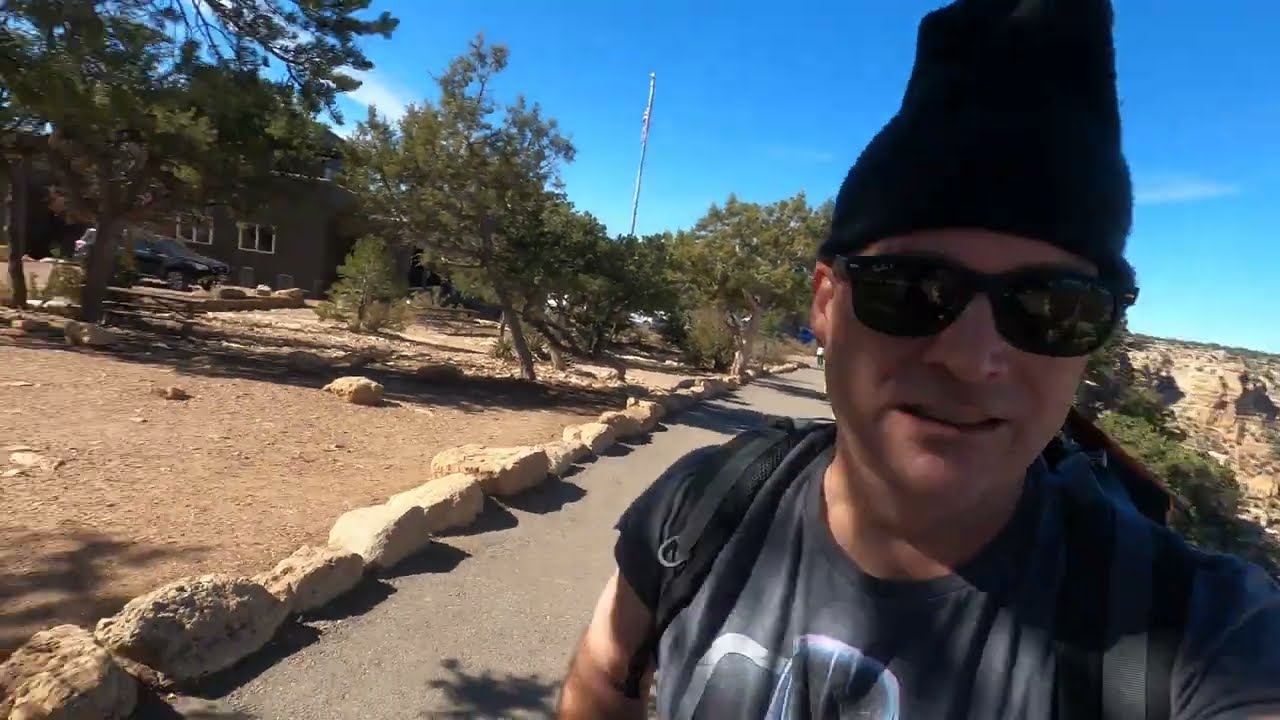In this wide, rectangular image, a white man estimated to be in his mid-30s is walking on a street. Only visible from the shoulders up, he is positioned on the right side of the frame, looking directly at the camera. He is dressed in a grayish-blue t-shirt with some text on it, a black beanie, and black sunglasses. He also wears a black and gray backpack. The outdoor setting suggests he is hiking or exploring nature. Behind him, starting from the bottom left corner and extending towards the right, is a gray paved road bordered by large tan rocks. Adjacent to these rocks is a neat dirt area with tall green trees. To the right of the man, a grayish-tan colored rock mountain and a light blue sky are visible. The right side of the image hints at a parking lot and some buildings. There are also signs of yards, a house, an automobile, and possibly a flagpole in the scene. It appears to be a sunny day with tree shadows on his face, indicating he is standing on a walkway edged with big rocks, possibly overlooking a canyon or at the edge of a path.